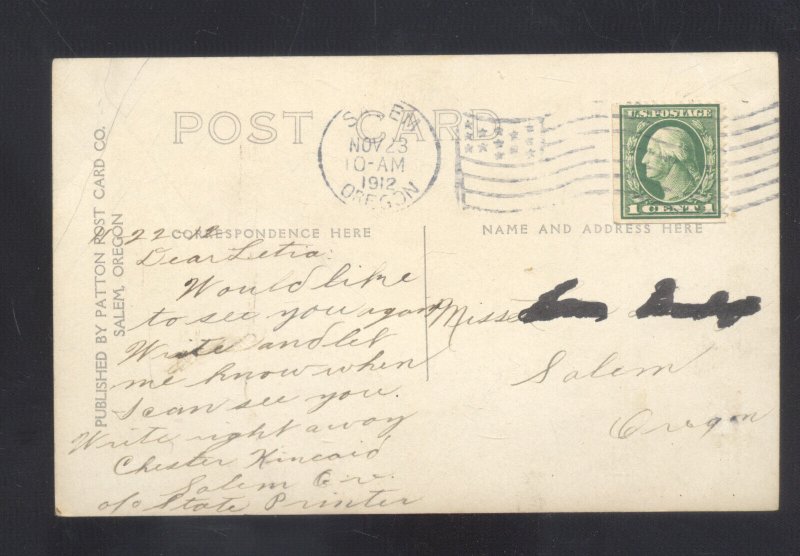This is an image of an old, faded postcard against a black background. The beige postcard features a green one-cent stamp in the far-right corner, depicting George Washington and marked with "US Postage." A round postmark, located in the middle, indicates it was processed at 10 a.m. on November 23rd, 1912, in Salem, Oregon. The header reads "POSTCARD," and partially legible writing can be seen across the back. The addressee's name is mostly obscured, but it is clear that the postcard is addressed to someone in Salem, Oregon.

In cursive writing, a message on the postcard reads: “Dear Letitia, would like to see you regarding Mrs. [unreadable]. Let me know when I can see you, right away. Chester Kincade, Salem, Oregon, in care of State Printer.” Additionally, parts of the postcard are watermarked, causing the ink to run and some details to be hard to decipher. The bottom mentions it was published by the Patton Ross Card Company in Salem, Oregon.